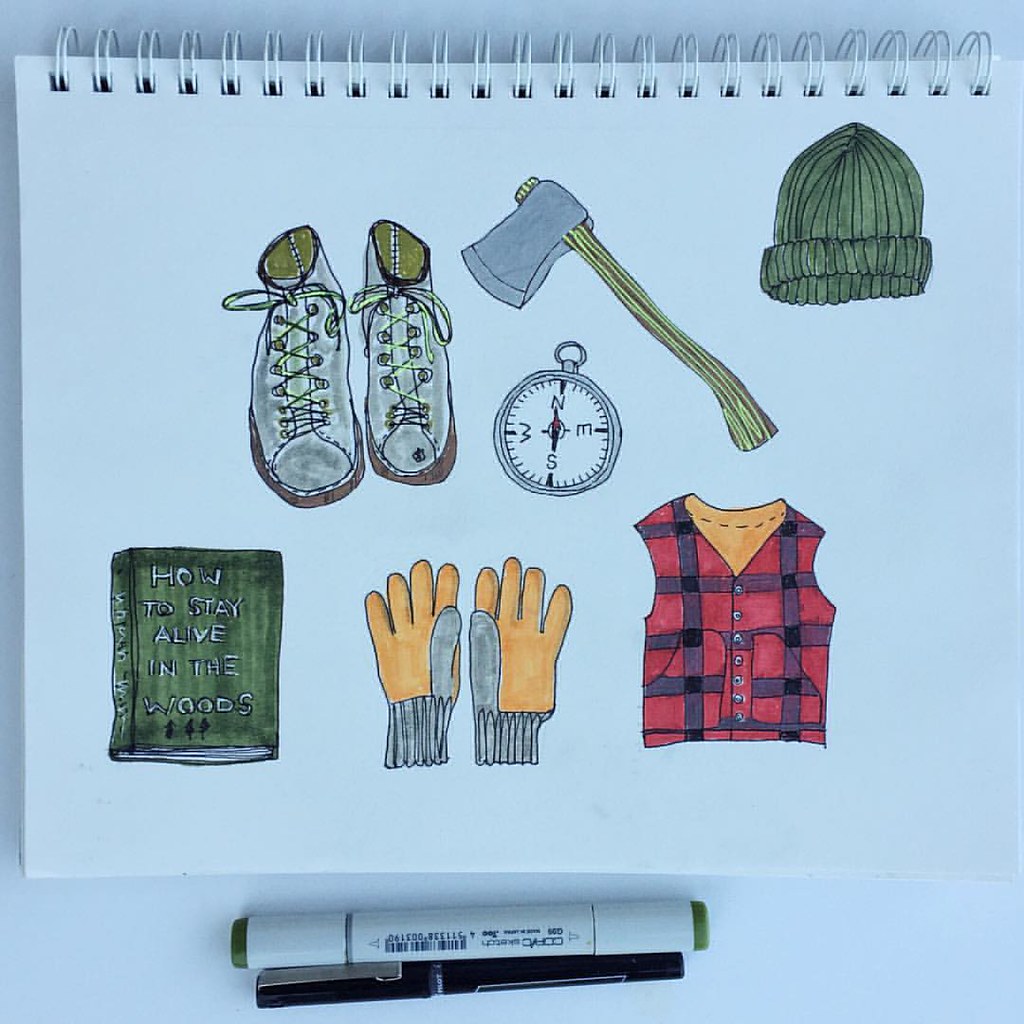This image showcases a detailed drawing of various survival and outdoor gear, meticulously sketched on a piece of white paper secured in a spiral-bound sketchbook. Prominently displayed on a white desk, the drawing features a collection of items typically associated with a woodsman or someone preparing for a wilderness adventure. 

In the upper right-hand corner, a green knit beanie is illustrated, paired closely with an axe to the left. Below the axe sits a compass, with its needle pointing north. Nearby, gray boots with their bright yellow laces tied in neat bows can be seen. In the bottom left corner, a hardcover book with a green cover reads "How to Stay Alive in the Woods," essential reading for any adventurer. Two pairs of orange gloves, featuring gray thumbs, are positioned to the right of the book, beside a red and black plaid vest typically worn by lumberjacks.

Accompanying the sketchbook at the bottom of the image are the drawing tools used: a dark green Copic marker and a high-quality black Pilot pen noted for its smooth gel ink. This collection of intricately drawn, woodsy-themed items underscores a narrative of preparation and survival in the great outdoors.